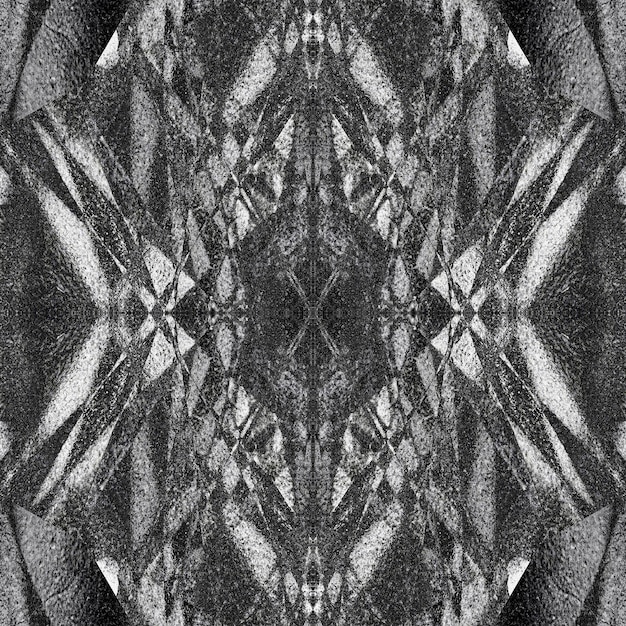The image showcases a highly detailed black and white painting reminiscent of a kaleidoscope's intricate patterns. Dominated by cascading, crystal-like triangular shapes, the artwork forms a captivating, symmetrical composition. At its center lies an eye-catching X shape formed by thick V shapes converging towards the middle, enhancing the image's symmetry. These shapes and designs, including gray circles and multiple intersecting triangles, create a mosaic-like, abstract aesthetic that feels both futuristic and somewhat out of focus. The top half of the image mirrors the bottom half, contributing to its hypnotic, almost AI-generated appearance. Predominantly monochromatic, this elaborate depiction evokes a sense of depth and complexity, inviting various interpretations.